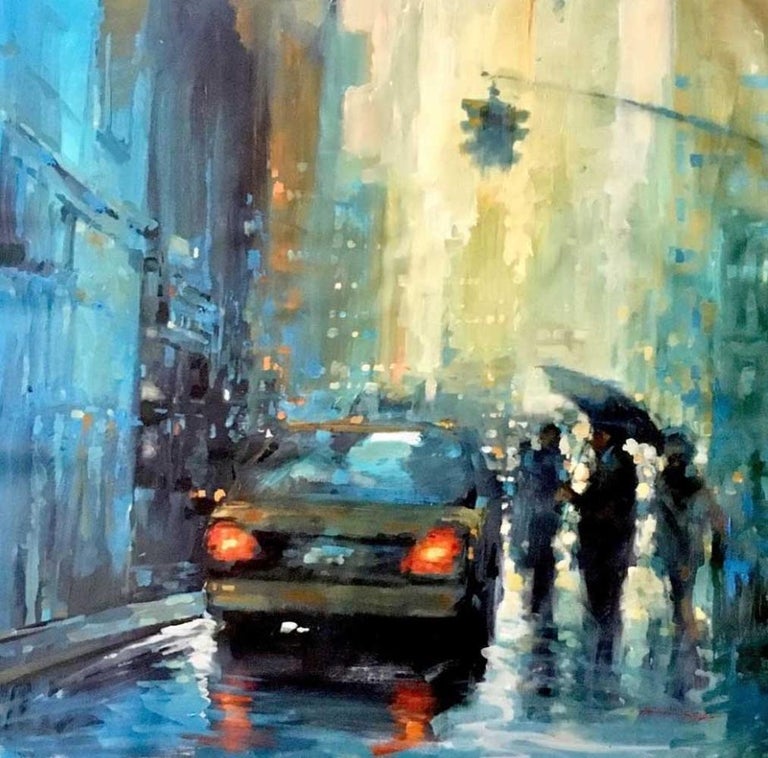The image depicts an abstract, oil painting of a rainy day on a bustling downtown city street. Blurry skyscrapers loom in the background, their details indistinguishable. In the foreground, a yellow vehicle, likely a taxi, sits with its brake lights glowing red, reflecting off the wet pavement. Four individuals stand in the rain, one of them holding an umbrella and wearing a black suit. Raindrops are visible, adding texture to the scene. At the top right, a street light mounted on a post suggests they are at an intersection. The streetlight casts a mix of red, green, and yellow hues, contributing to the lively yet somewhat somber ambiance. The left side of the painting features a building, with the overall scene rendered in a palette dominated by blues, yellows, and blacks. The painting captures the busy, rainy atmosphere of the city through a blend of abstract forms and vivid colors.